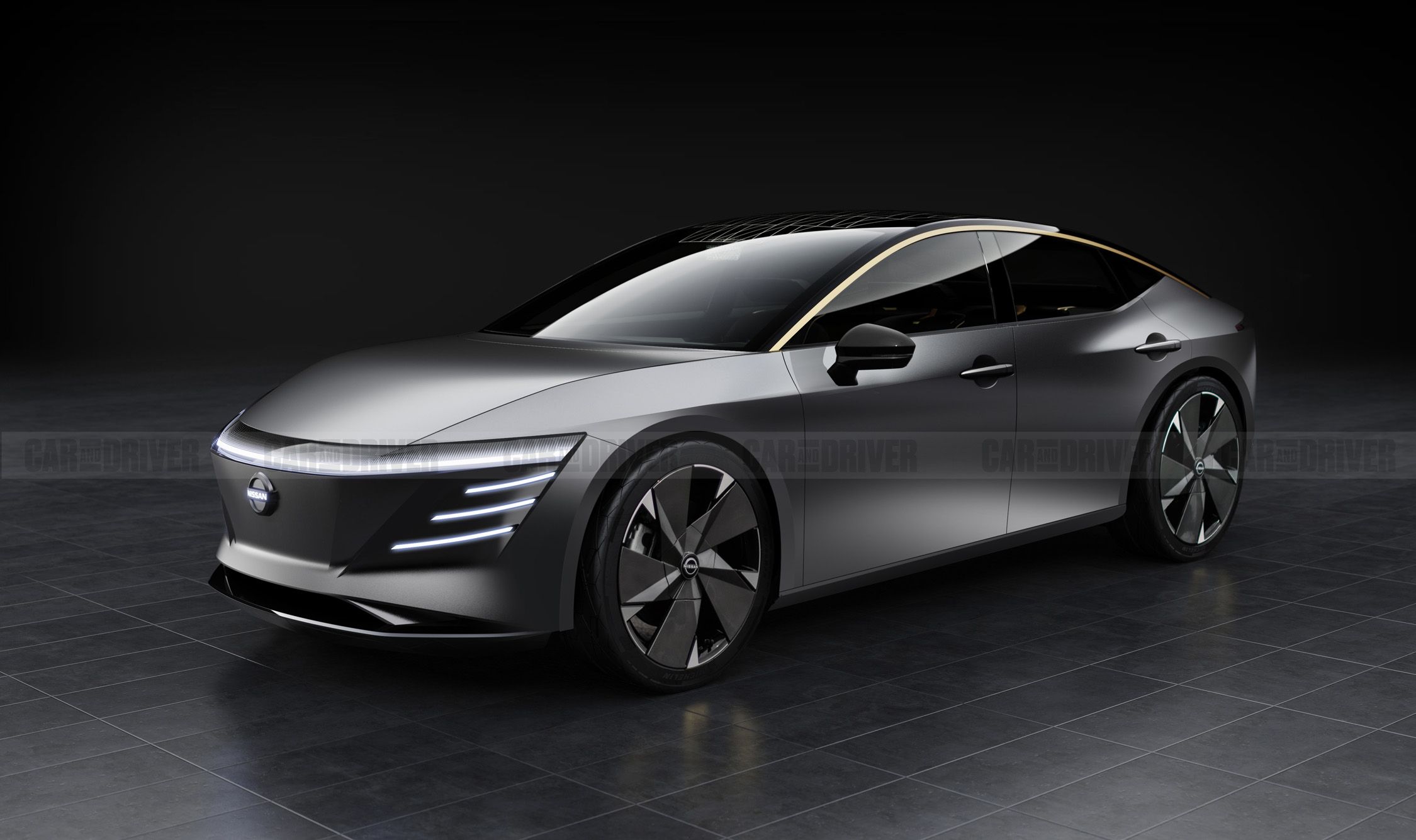The image displays a side view of a futuristic-style Nissan Maxima with a sleek, gunmetal gray, metallic finish. This four-door sedan features a gold outline running from the bottom of the windshield to the back window along the driver's side. The car is adorned with shiny silver wheels and large, elegant hubcaps. The front of the vehicle showcases an angular design with a thick grille prominently displaying the Nissan logo. The headlights are a distinctive, continuous LED light bar that wraps around the hood, accompanied by three thin LED lines beneath the main headlights. The car sits on a reflective black tiled floor, with the lighting meticulously set up to accentuate its shiny, futuristic appearance. The background is entirely black, creating a stark contrast that emphasizes the car's reflective surfaces. There is a faint watermark across the middle of the image, reading "Car and Driver," giving it a professional, showroom quality.